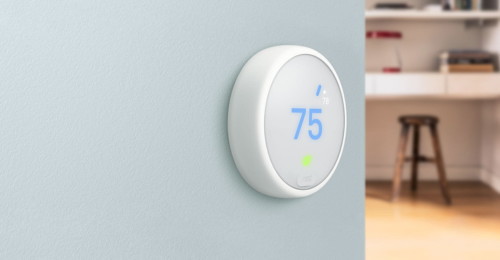Cropped in a landscape orientation, this interior scene prominently features a thermostat mounted on a light blue wall that occupies two-thirds of the image on the left. The thermostat is angled towards the upper right corner and has a white rim with a white display showing a blue "75" and a small green LED indicator below it. On the right side of the image, there's a glimpse of the room which includes a brown wooden stool next to a white countertop with a white shelf above it. Various objects are placed both on the countertop and the shelves. The wooden floor, gleaming due to the light source from the left, shows a bright spot in the lower left portion while the bottom right corner remains darker.